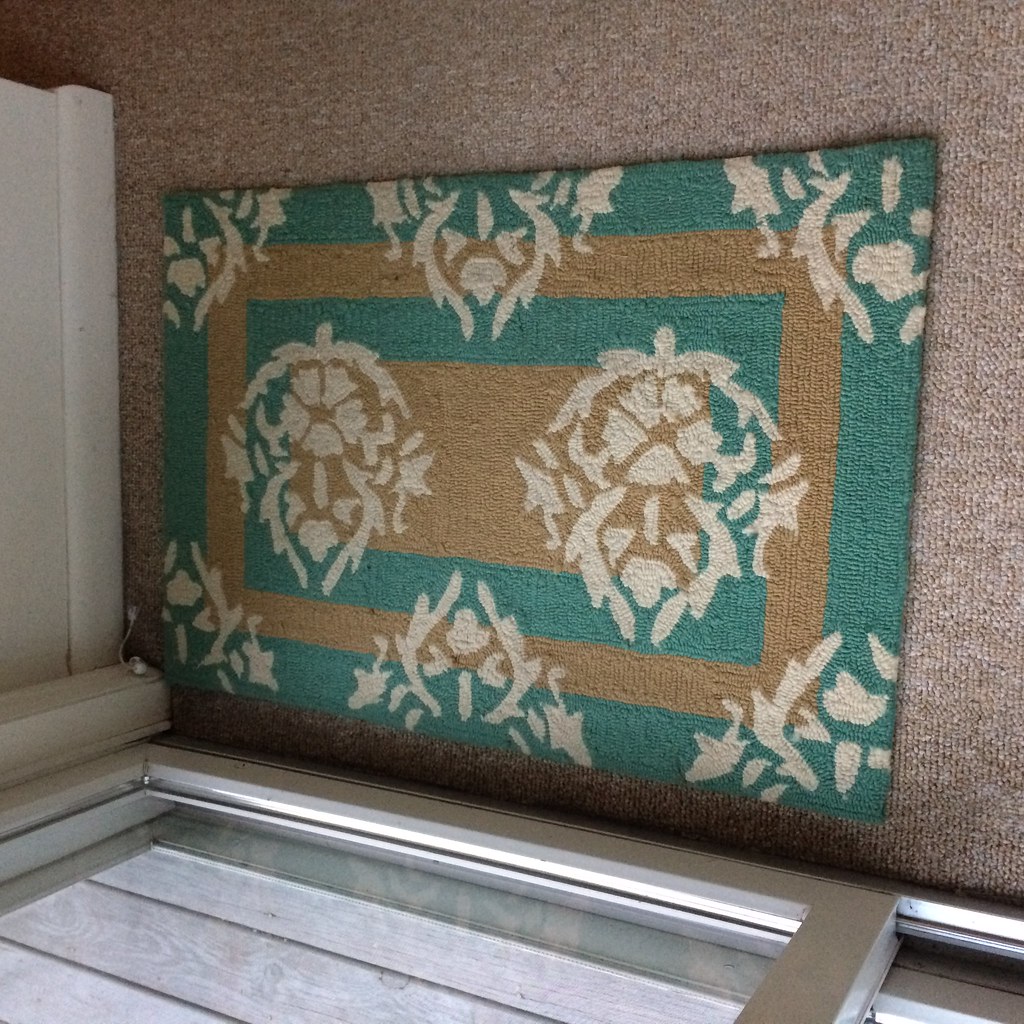This photograph, taken from an overhead angle, captures an interior space featuring a layered flooring arrangement. Dominating the image is a small, rectangular throw rug, approximately three feet by four feet, placed on top of a larger, tweed-style brown carpet. The throw rug itself is an intricate composition of blue-green and beige rectangles, framed by repeated patterns of similar colors. The central area of the rug integrates a large dark gold rectangle adorned with abstract white designs, which resemble either pine cones or abstract faces. The bottom of the image reveals a gray deck through the partially visible aluminum frame of a sliding glass door, suggesting that the doormat functions as a transition point for wiping feet before stepping onto the actual carpet.